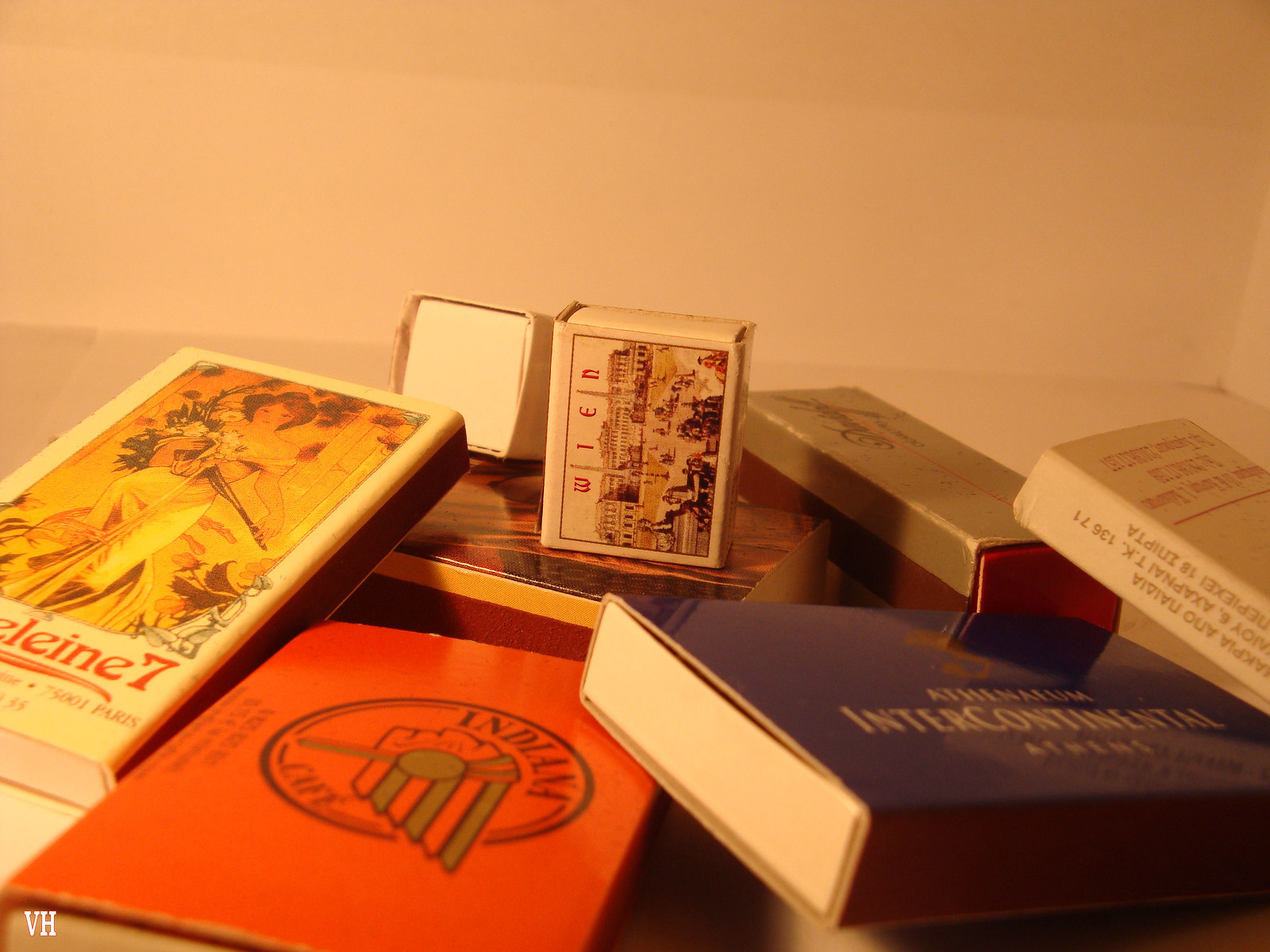This image showcases an eclectic assortment of eight matchboxes, artfully arranged on a peach-colored backdrop with a slight glimpse of a wooden table or ledge along the bottom edge. Each matchbox boasts its own unique design and color scheme, lending a vibrant and nostalgic ambiance to the scene. 

Prominently displayed in the collection is a small matchbox standing on its end, labeled "WIEN" with an intricate depiction of a large building adorned with two tall chimneys and a bustling courtyard below, reminiscent of an English setting. Adjacent to this matchbox is a square box nestled within a sleeve. Another notable matchbox, partially visible, reads "E-L-E-I-N-E 7" and features a detailed illustration of a woman in a dress holding a bouquet, rendered in warm orange and yellow tones.

An orange-red matchbox inscribed with "Indiana Q" exhibits an Indian head with a headdress, adding a touch of cultural flair. Directly in front of this, a dark blue or black matchbox stands out with the words "Intercontinental Athens."

Other matchboxes in the arrangement include a white one with gold lettering, paired with red text and an underline, potentially spelling "Ananasia." Additionally, there's a box with a dark-colored image and striped design, possibly of someone in a tan suit. One matchbox on its side and another square box further enrich the diverse assembly.

Together, these matchboxes create a visually engaging tableau of varied designs and hues, evoking a sense of curiosity and nostalgia.